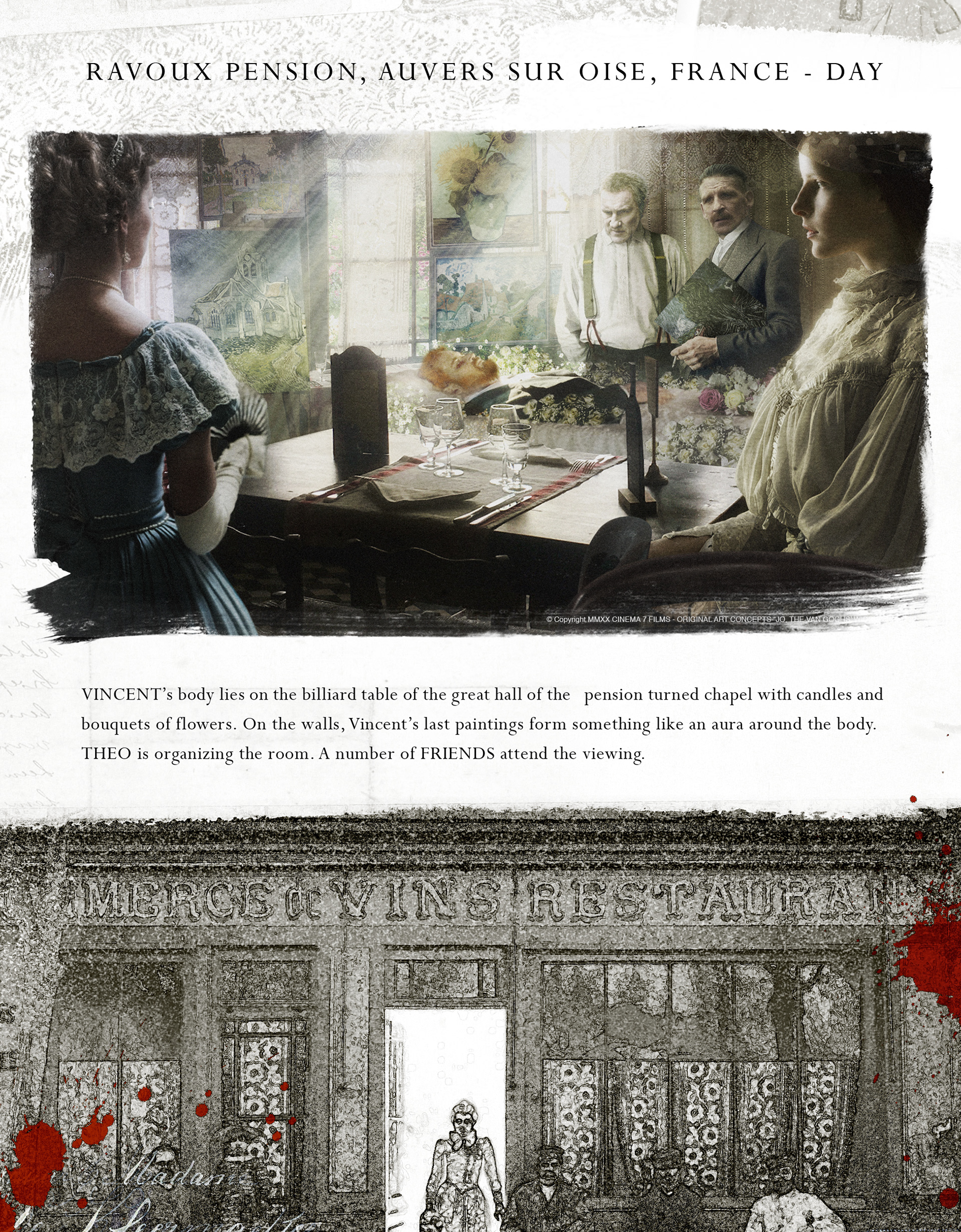The image is divided into two panels. The top panel appears to be a detailed oil painting or an artist's rendering depicting a somber interior scene, presumably a funeral. In this scene, a body, believed to be Vincent van Gogh, lies in state on a coffin or a makeshift bier, set upon a billiard table in the great hall of a pension-turned-chapel. The setting is adorned with candles and bouquets of flowers, and Vincent’s last paintings form an almost ethereal aura around the body, enhancing the scene's poignancy. Two women donning ornate, possibly 1800s-era clothing, stand on either side of the body, one holding a fan. Two men are also present, with one identified as Theo, who seems to be organizing the room. A number of friends are in attendance, paying their respects.

The bottom panel features a contrasting black-and-white image of a building facade with a storefront sign that reads “Merck's and Vin's Restaurant.” The scene includes splotches of red, suggestive of blood, adding a dramatic element. Text in a foreign language appears at the top of this panel, reading "Ravot Pension, Averse Sir Oise, France Day," situating the scene in an old French setting.